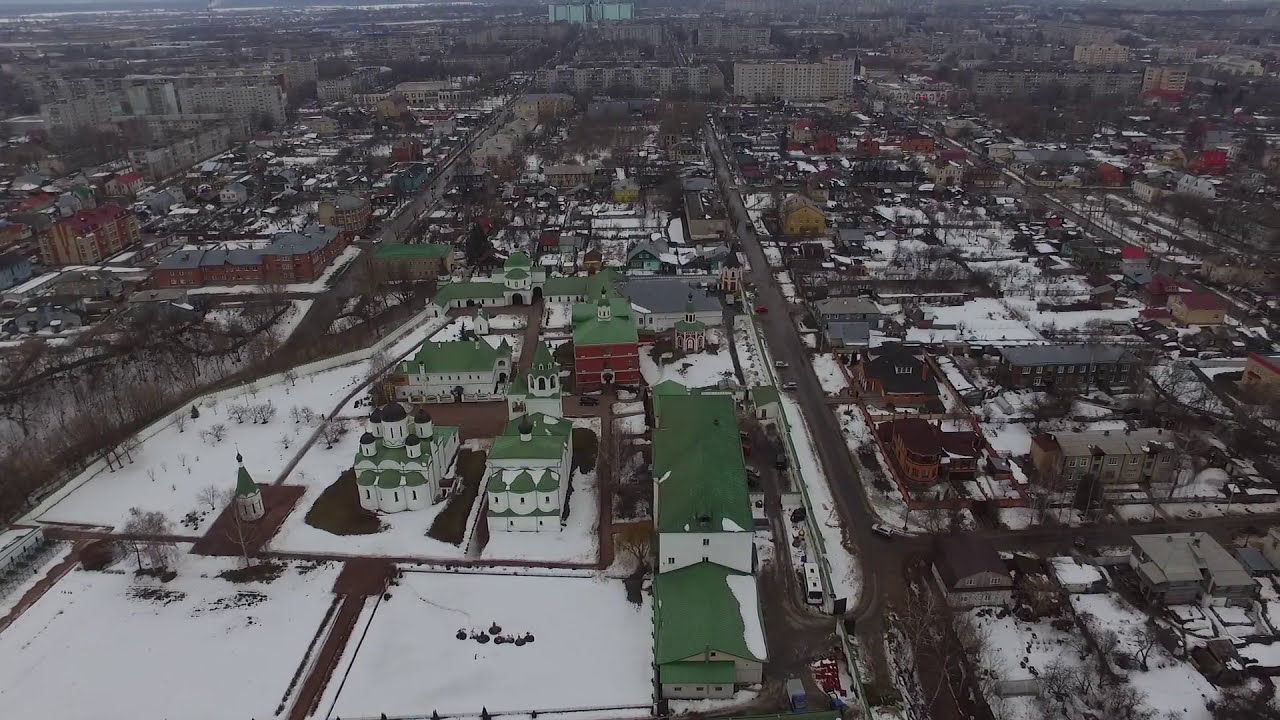This color photograph is a detailed aerial view of a snow-covered town captured in landscape orientation, likely by a drone. The ground is blanketed in snow, except for the clear roads where cars are visible driving throughout the town. Dominating the foreground are several large, white-sided buildings with green roofs, evoking an old, almost Russian architectural style. These buildings are clustered together, forming a cohesive complex. Surrounding these are smaller neighborhoods with buildings of varying types, including brick structures with black and gray roofs.

A prominent gray street cuts diagonally from the bottom right of the image towards the horizon at the top, dividing the town. To the left in the foreground, there appears to be housing with green roofs and large snowy fields in front. Near the center, a notable building with a spire—potentially a chapel—stands out, also surrounded by snowy fields. In the background, the town extends with clusters of houses packed closely together and larger commercial buildings that resemble motels or hotels. The wintry scene is devoid of much foliage, with patches of snow covering roofs and yards, providing a stark, realistic depiction of the town in winter.